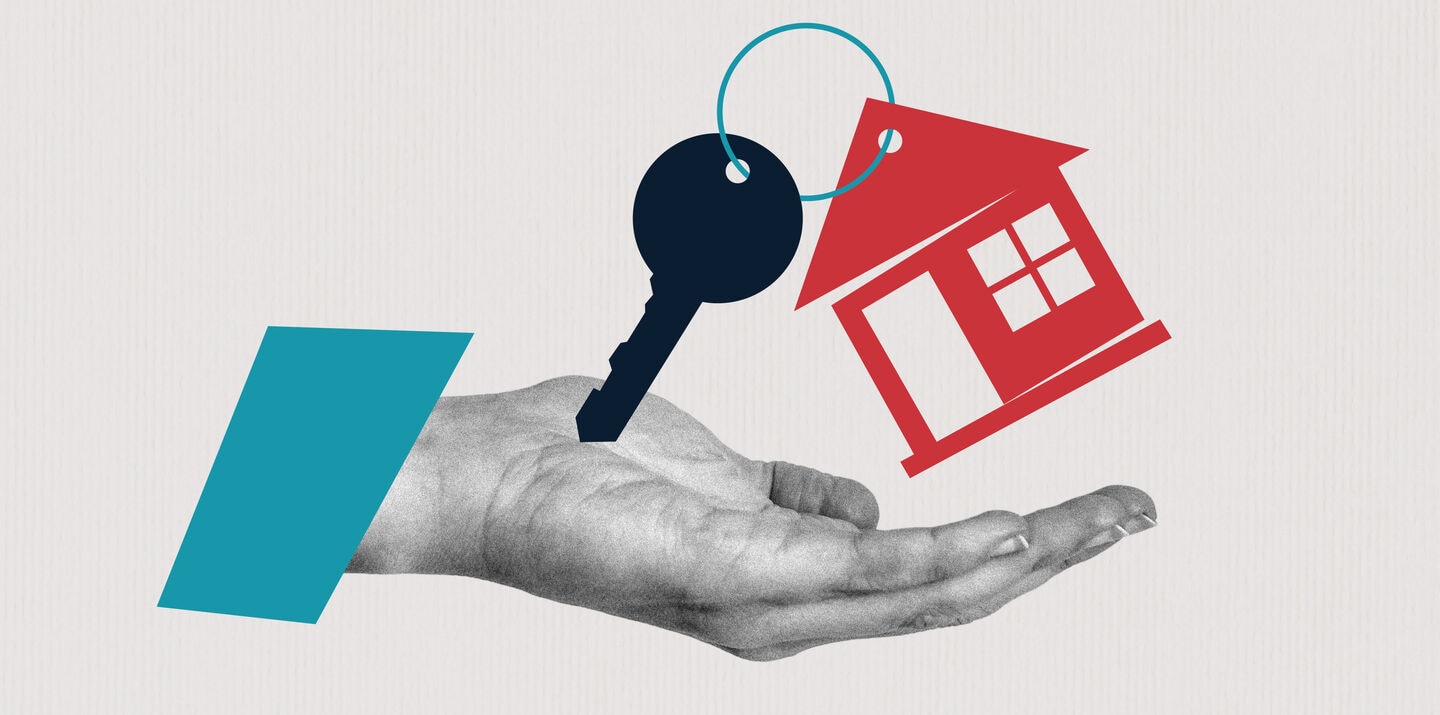The image is a close-up graphic of a Caucasian person's left hand, which is stylized in black and white, with the palm facing forward and laying flat, appearing to be cupped slightly as if in a gesture to receive something. A teal blue, cartoon-like cuff adorns the person's wrist, transitioning into a rectangular turquoise shape. In the center of the palm, there is a vivid, simple illustration featuring a black key attached to a key ring. The key ring is the same teal color as the cuff and loops through the top of a red house, positioned to the side of the key. The house is drawn with a triangular roof and a rectangular body, complete with four small square windows and a small rectangular door, suggesting a typical house structure. The background is blank, making the graphic elements and the central theme of home and ownership stand out, possibly indicating a connection to real estate or home services.